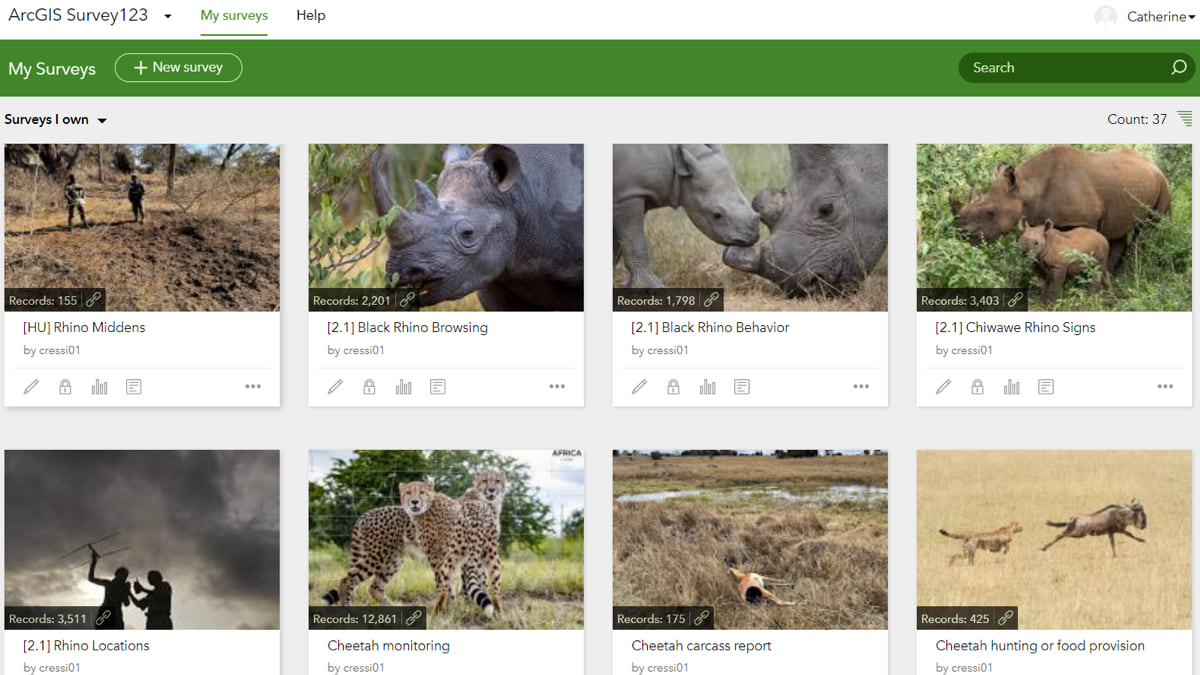A screenshot from the ARCGIS Survey123 application showcases a variety of animal-related survey entries. At the top of the interface, we see options such as "My Surveys," "Help," and a prominently displayed green tab labeled "My Surveys." There is a plus sign to create new surveys and a search bar on the right for easy navigation.

The page displays several thumbnail images organized into two rows of four. The first row features:
1. An image depicting two individuals in a desert environment with the caption "Rhino Middens."
2. A photograph of a rhino labeled "Black Rhino Browsing."
3. A picture displaying a baby rhino alongside an adult rhino, captioned "Black Rhino Behavior."
4. An image of another baby rhino with a larger rhino, labeled "Chihuahua Rhino Signs."

The second row contains:
1. A photo taken from a lower angle of two people standing under a dark sky, seemingly carrying sticks, with the caption "Rhino Locations."
2. An image of two cheetahs labeled "Cheetah Monitoring."
3. A disturbing picture of an animal, appearing to have collapsed, titled "Cheetah Caress Report."
4. An action shot of a cheetah chasing another animal, possibly a goat, under the caption "Cheetah Hunting or Food Provision."

This detailed visual summary provides a glimpse into various wildlife surveys focusing on rhinos and cheetahs, complete with specific behaviors and environmental contexts.